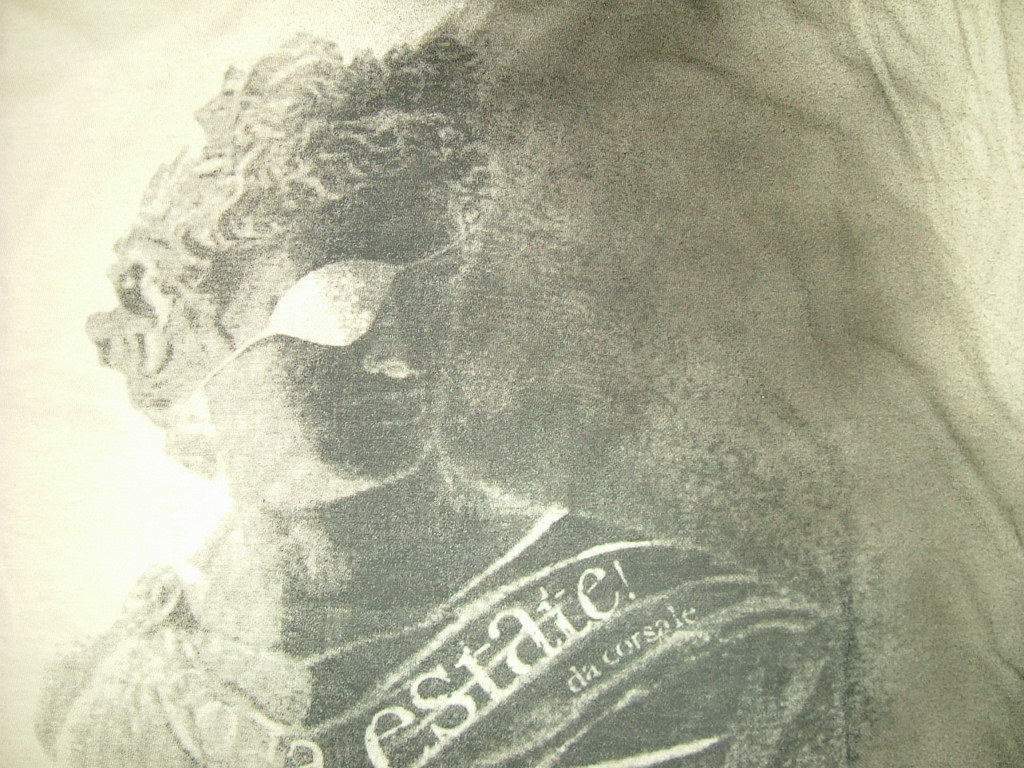The image appears to be a meticulous pencil drawing of a figure that closely resembles an ancient Greek statue. The figure features a distinctive eyepatch over his right eye and is gazing to his left. The details capture the essence of classical sculpture, characterized by curly hair, a prominent Roman-style nose, and subtly veiled lips. One can discern intricate details like the outline of the eye across the chest. The figure is adorned in what seems to be the upper part of a traditional toga. Inscribed on the figure's left side are the words "Estate da Corsale," with "Estate" placed above "Corsale." On the right side, some letters are visible but not clearly legible. The background is shaded, giving the impression that the figure is casting a shadow on a textured wall that resembles a sheet. The lighting comes from the figure’s right, enhancing the shadows and adding depth to the composition. The entire artwork predominantly uses shades of black, tan, and white.